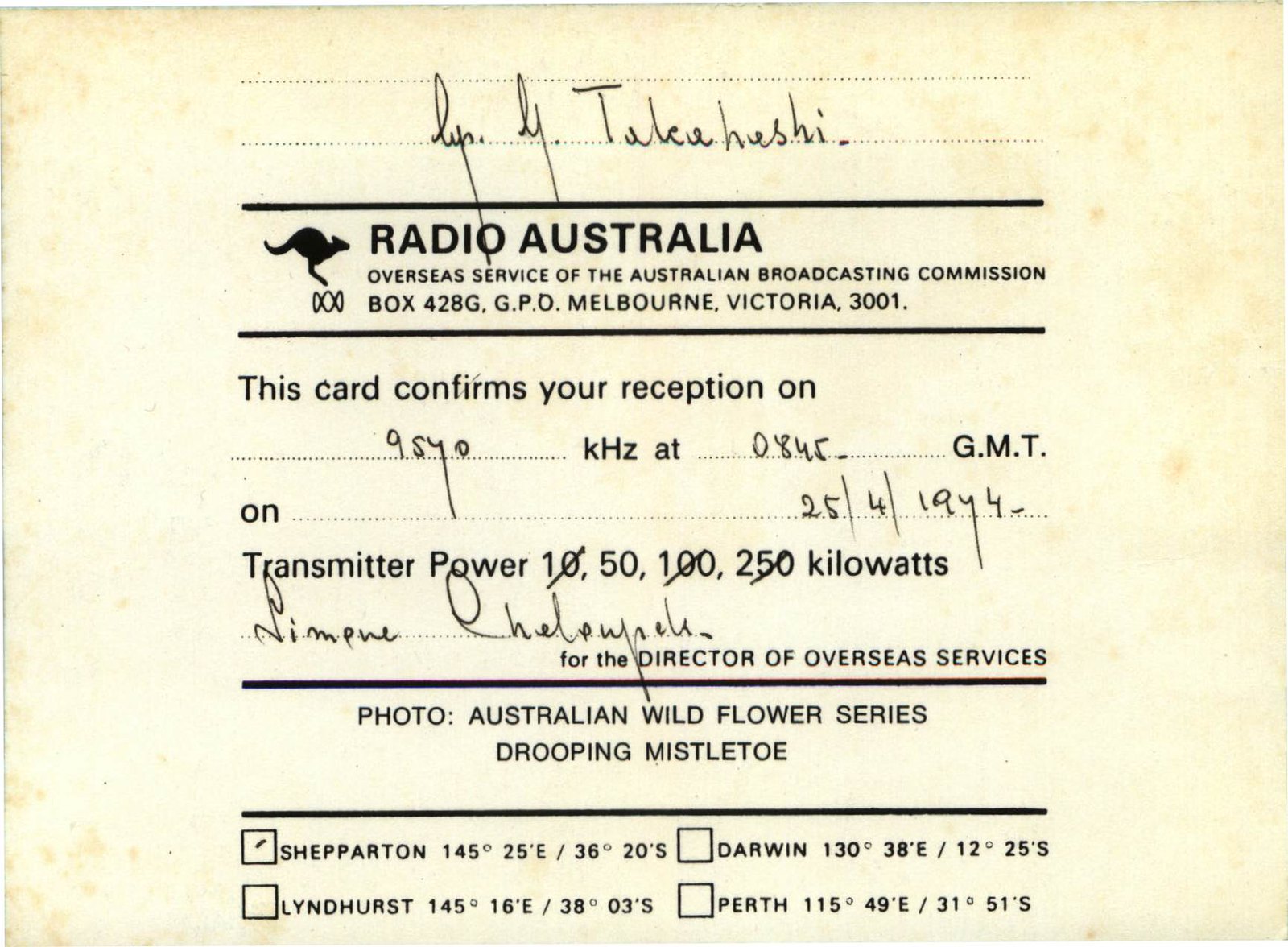The image depicts an old, yellowing radio confirmation card, weathered with age and dotted with spots. At the very top is an indistinct signature, which appears to be signed by someone named Takahashi. Beneath this signature is a small icon of a kangaroo, accompanied by the text: "Radio Australia, Overseas Service of the Australian Broadcasting Commission, Box 428G, GPO, Melbourne, Victoria, 3001."

Following this, the card states: "This card confirms your reception on 9540 kilohertz at 0845 GMT on 25th April 1944." The transmitter power is indicated as 50 kilowatts, with options for 10, 100, and 250 kilowatts noticeably crossed out. Below this confirmation, there is a printed name on a dotted line, representing the Director of Overseas Services.

At the bottom portion of the card, the text indicates a series featuring Australian wildflowers, specifically the "Drooping Mistletoe." Also visible are location coordinates with check boxes, indicating a specific location marked as "Sepperton, 145 degrees, 25 East / 36 degrees, 20 South." The layout points towards a meticulous record of a radio reception, likely for administrative purposes within the broadcasting service.